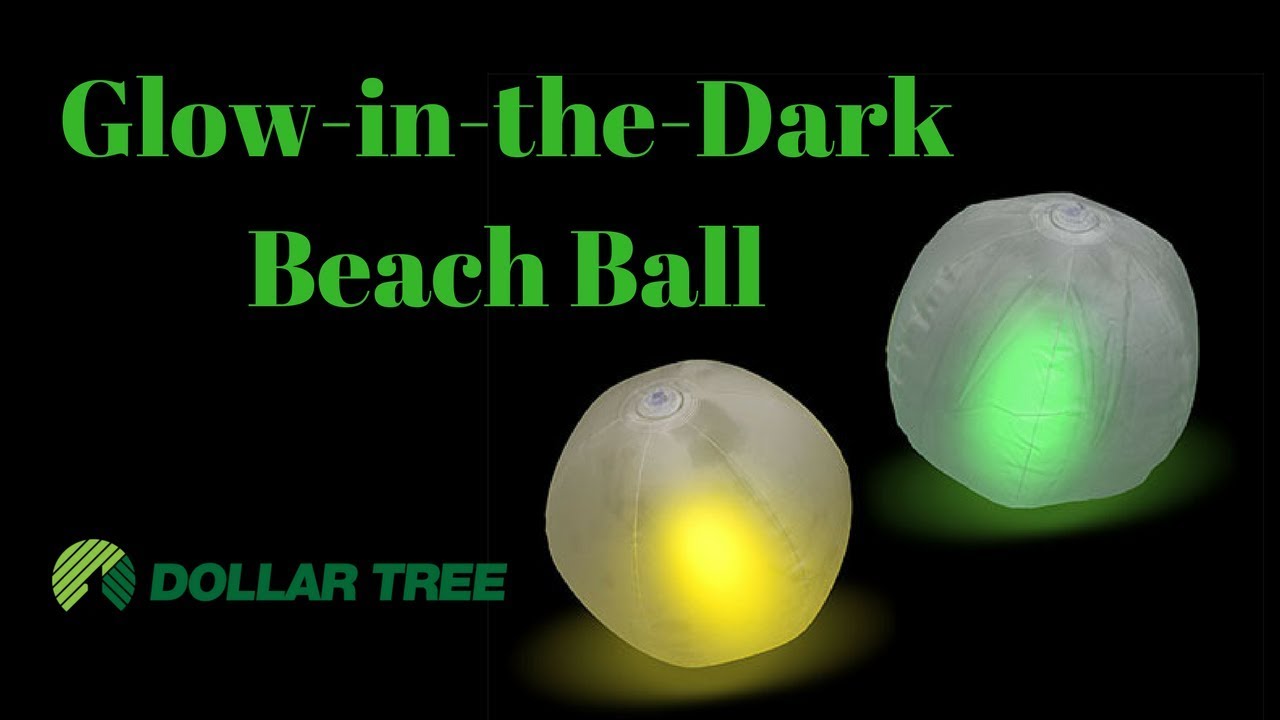This advertisement for a product features a black background with striking fluorescent green text in the top left and center that reads "glow in the dark beach ball." In the bottom left-hand corner, the Dollar Tree logo is prominently displayed, featuring a circular icon with light yellow and dark green stripes and the words "Dollar Tree" in lime green lettering. To the right side of the image, two translucent, slightly cloudy, inflatable beach balls are showcased. The ball on the left displays a bright glowing yellow light inside, while the ball on the right contains a bright glowing green light. Each ball is mostly clear, with the illumination localized within the center. Inflatable tabs are visible on the top of each beach ball, emphasizing their functionality and design.